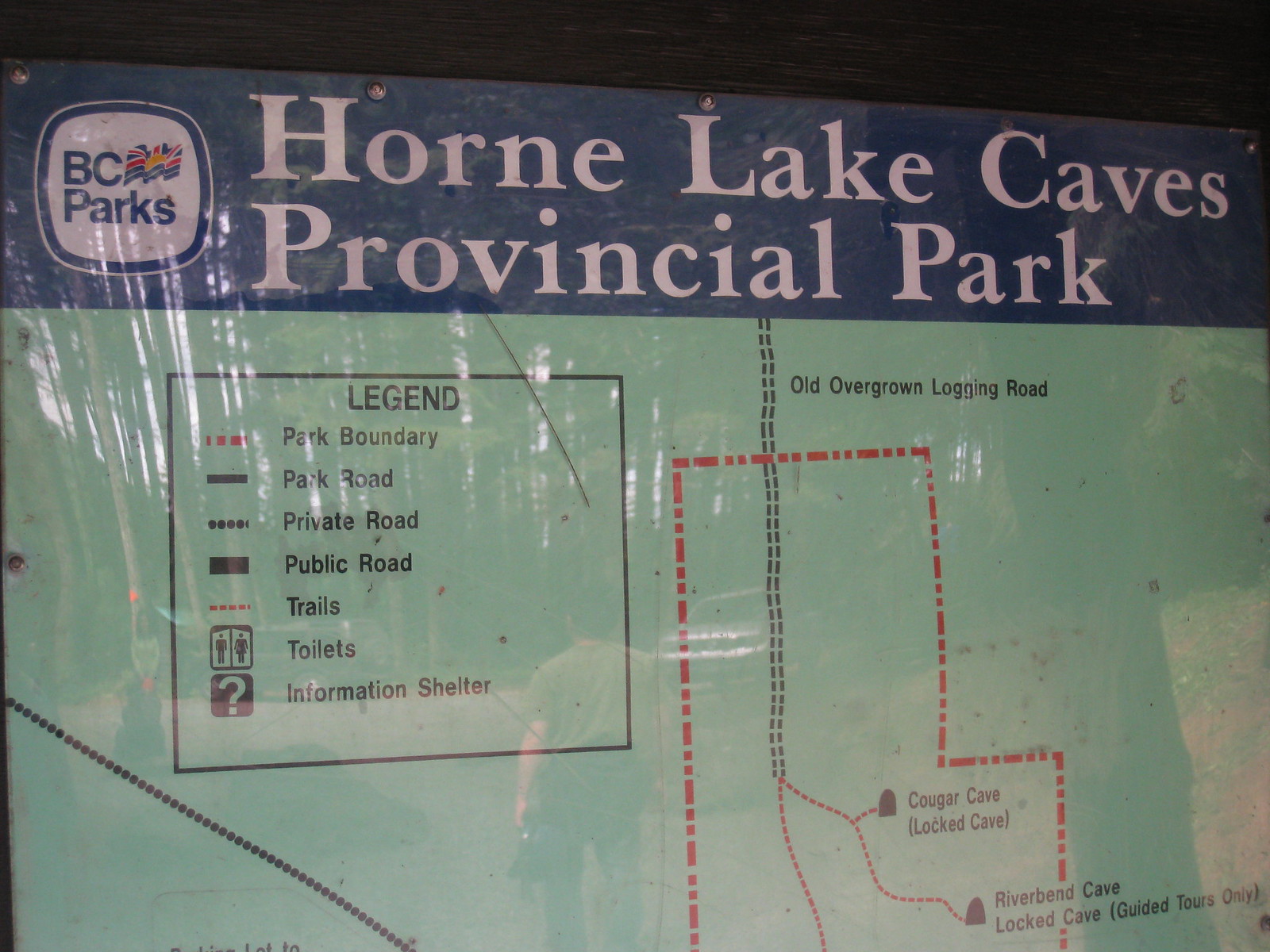The image features a detailed sign for Horn Lake Caves Provincial Park, set against a green background with a blue strip at the top containing white text. Prominently displayed at the top is "Horn Lake Caves Provincial Park," alongside a circular BC Parks logo with a flag inside. The sign includes a legend that defines various identifiers: red dots for the Park Boundary, a solid black line for the Park Road, a dotted line for the Private Road, and a larger rectangle indicating the Public Road. It also marks Trails with red dots, shows icons for Toilets with figures of a man and a woman, an Information Center with a question mark, and notes an Old Overgrown Logging Road. The sign showcases a map highlighting features such as Cougar Cave, Riverbend Cave, and Locked Cave, noting that the latter two can only be accessed through guided tours. The overall map layout is organized horizontally within a rectangular frame, providing a clear visual guide to the park's key locations and amenities.